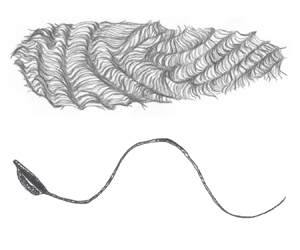This image features a detailed sketch on a white background with two distinct parts. The top section depicts a fur-like structure with a striped, grooved pattern, resembling a sweater knit together with thick ropes. This section transitions from smaller to larger in width as it moves from right to left and is illustrated in varying shades of gray, akin to pencil or charcoal strokes.

Below this knitted pattern, there is a depiction of what appears to be a unicellular organism, possibly a sperm cell, characterized by a dark, solid charcoal gray head, and a wiggly tail or cilium. This squiggly line, darker than the top section, traverses from right to left, curling downwards before rising to a peak and descending again. The organism's tail appears intricate, giving the impression of a flexible, dynamic shape. Both parts of the drawing showcase the artist's precision and shading techniques, highlighting the biological theme and magnified cellular structures.